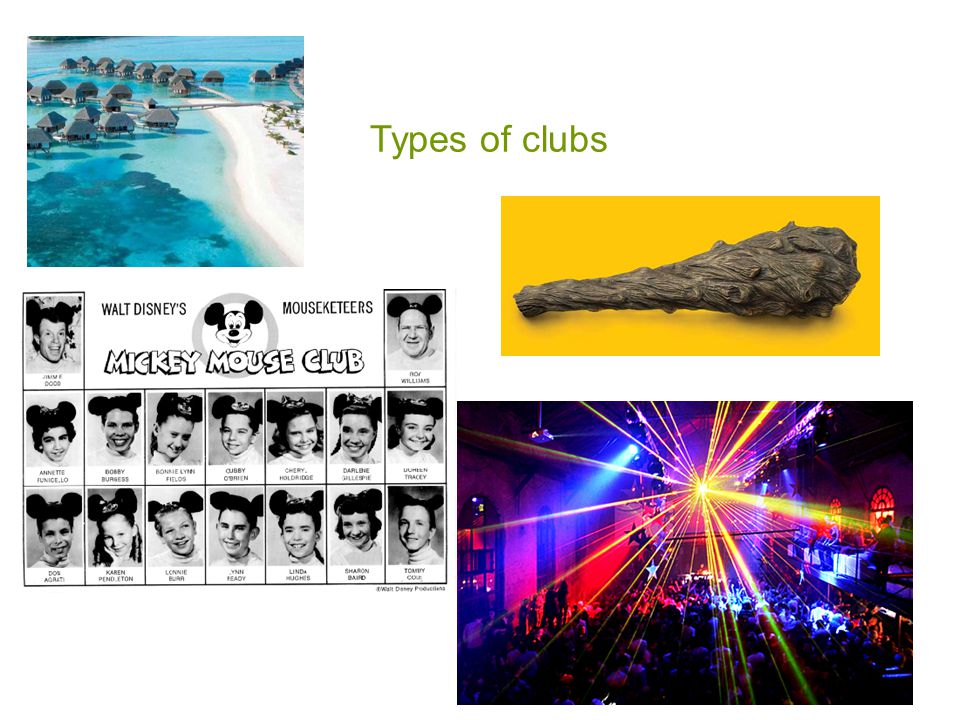The image is a collage titled "Types of Clubs," written in green font with the word "Types" capitalized. This title is placed centrally against a white background. Surrounding the title are four distinct pictures:

- The top-left image showcases a serene coastal ocean environment featuring numerous small residences above water, suggestive of a luxurious and tranquil tropical retreat.
- Below it, the bottom-left image in black and white depicts the original Mickey Mouse Club, showing children and adults donning iconic Mickey Mouse ears.
- To the right of the title, the top-right picture displays an ancient-looking wooden club with a small handle and a broad end, set against a yellow backdrop.
- Lastly, the bottom-right image captures a vibrant nightclub scene, complete with a crowded dance floor and flashing, multicolored lights, epitomizing modern nightlife.